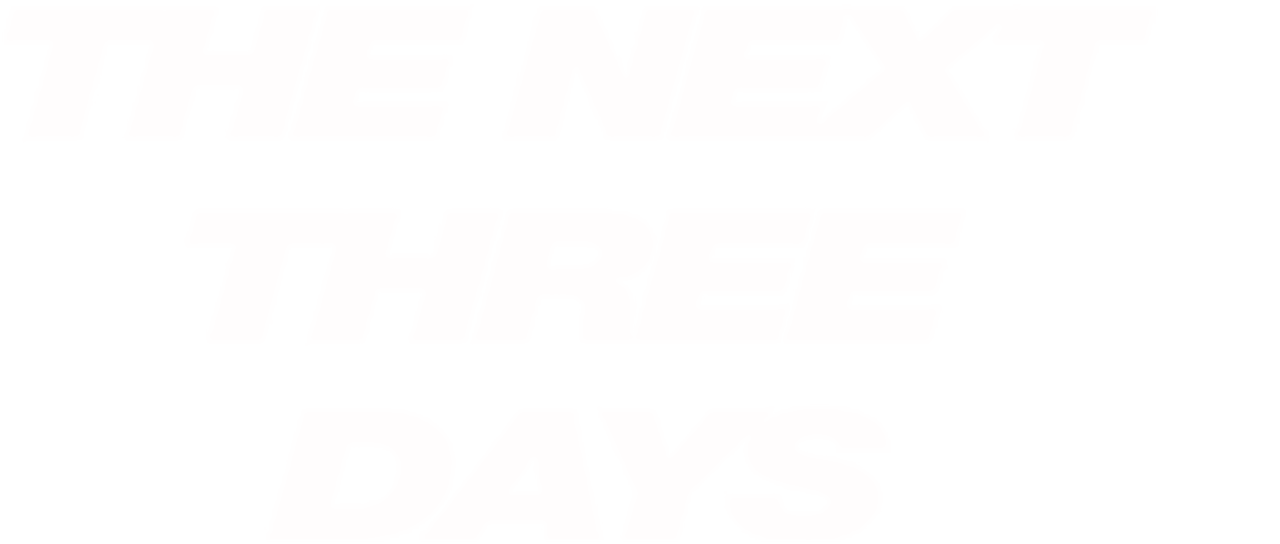The image in question appears to be a completely blank, white canvas. Despite multiple attempts to reload and view the image across different browsers and devices, no content has become visible. Users have reported waiting for extended periods, clearing cookies, and even troubleshooting with different system configurations, including using a Chrome browser on an M1 Macintosh chip. However, all efforts to reveal any objects or details in the image have been fruitless. Thus, the canvas remains entirely white and blank.